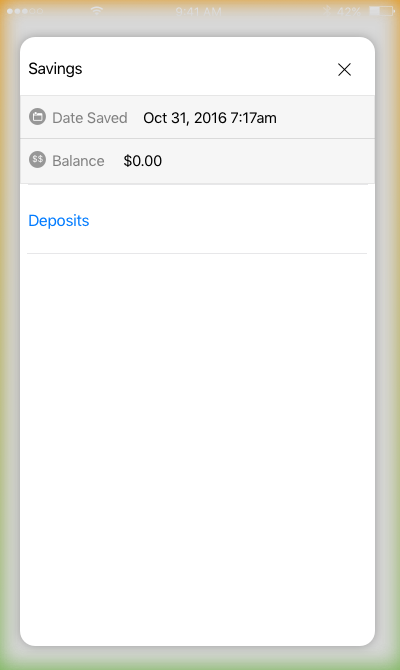This is a detailed screenshot of a mobile banking application window, titled "Savings," visible at both the top and top-left corners. The top-right corner features a close icon represented by a black cross. Beneath the title bar, two entries are displayed under light grey tabs. 

The first entry, labeled "Date Saved" in grey text, shows the date and time as "October 31st, 2016 at 7:17 a.m." in black text. The second entry, labeled "Balance" in grey text, displays the account balance as "Zero dollars and zero cents" in black text. Below these entries, the word "Deposits" is in blue text followed by a thin grey line.

The white window housing this information is outlined in a grey border. The background of the phone screen, partially visible behind the white window, shows additional elements. In the top-left corner, there are five dots, with three filled in white, alongside a faintly visible Wi-Fi symbol. The center of the screen displays the current time, "9:41 a.m." On the extreme right, both the Bluetooth icon and the battery charge level, indicating 42%, are visible.